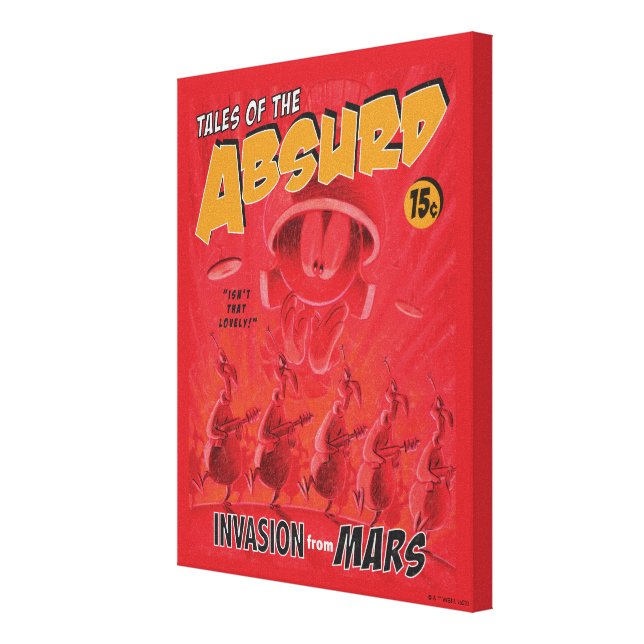The image depicts a cover, likely of a book or DVD, titled "Tales of the Absurd." The overall background is red, with the title "Tales of the Absurd" prominently featured in bold text. The words "Tales of the" are in white with black outlines, while "Absurd" is in a dark, dull yellow with white outlines and black shadows. On the cover, there is a red image of Marvin the Martian, a character from Warner Brothers' Looney Tunes. Marvin is depicted clapping his hands, which are drawn in a cartoonish style resembling gloves. To the left of Marvin, in black text with quotation marks, it reads, "Isn't That Lovely?" In the upper right corner of the image, a small yellow circle contains the price "15 cents" in black text. Below Marvin, there is a marching formation of bird-like creatures, each equipped with laser ray guns. These birds have beaks, small heads with feathers, white eyes, and stand upright with arms and legs. Beneath this scene, the text reads "Invasion from Mars," with "Invasion" in black with white outlines, "from" in white, and "Mars" in black with white outlines. The image appears against a plain white background with no visible borders, making it prominent and eye-catching.